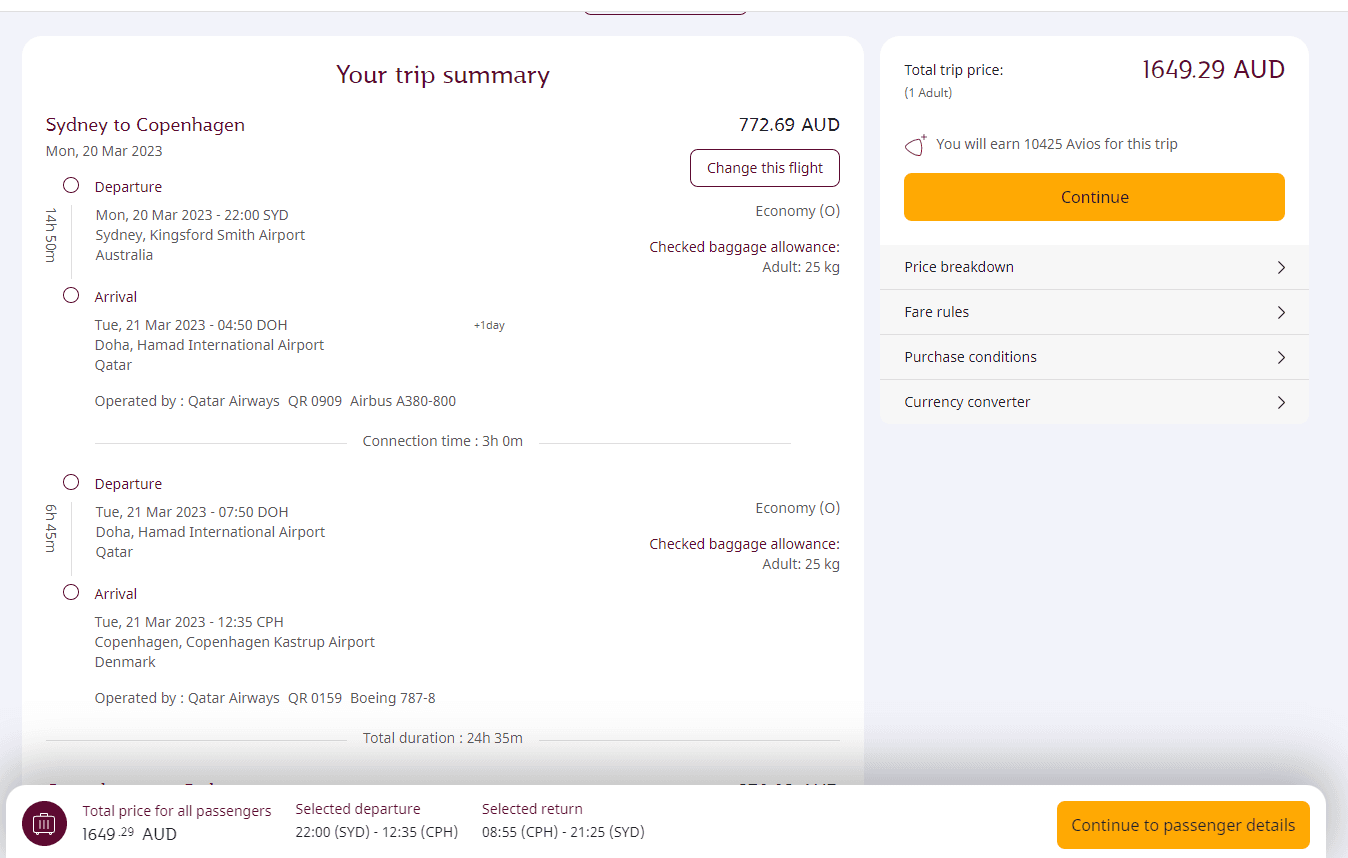This image resembles a flight booking website showcasing a detailed trip itinerary. The layout consists of two sections: a broader left section titled "Your Trip Summary" and a narrower right section labeled "Total Trip Price." 

In the "Your Trip Summary" section, it details the flight from Sydney to Copenhagen. The journey begins on Monday, March 20th, 2023, departing from Sydney Kingsford Smith Airport, Australia. The flight is operated by Qatar Airways and has a stopover at Doha Hamad International Airport, Qatar, arriving on Tuesday, March 21st, 2023. 

The "Total Trip Price" section to the right is concise, displaying the total cost for the trip, which is $1,649.29 AUD. 

This image effectively provides a clear and comprehensive overview of the flight itinerary and cost for a trip from Sydney to Copenhagen.